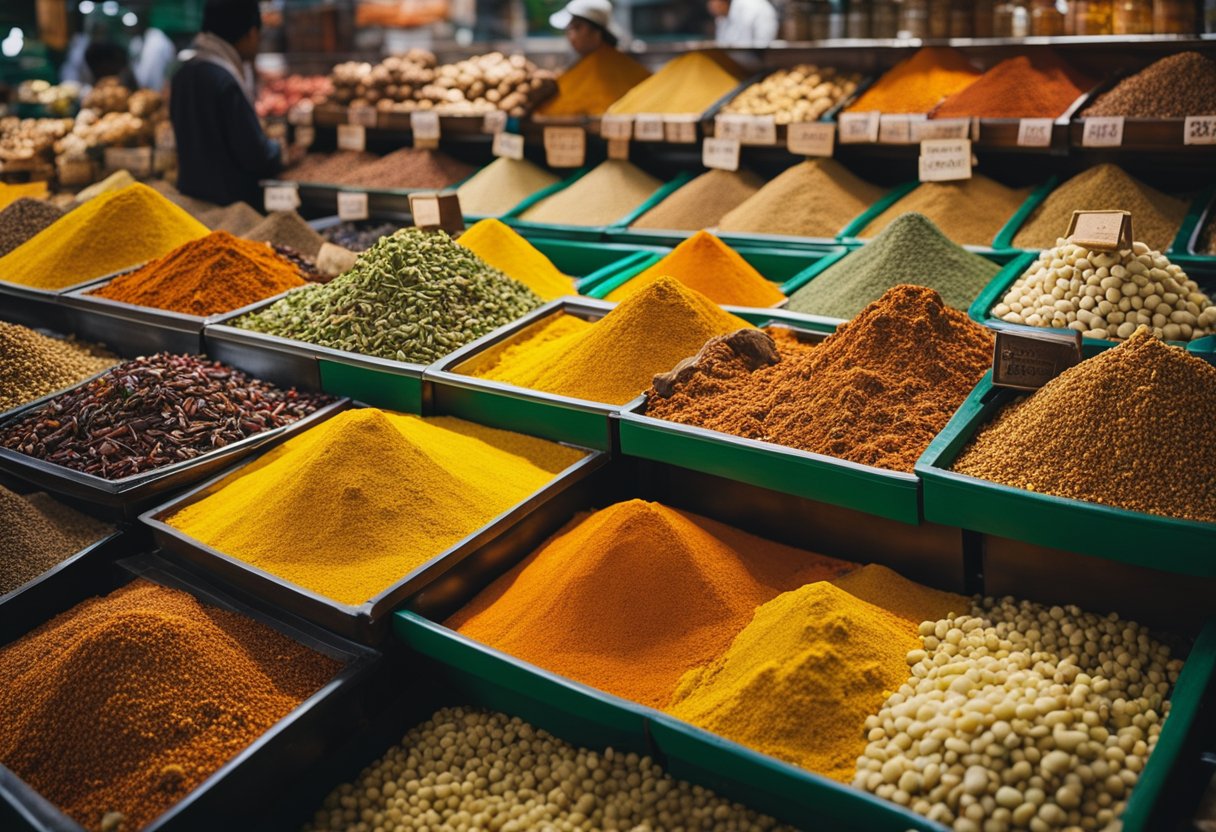This photograph captures the vibrant scene of an indoor spice market, likely of Indian origin, centered on a bustling spice stall. The stall features a myriad of spices presented in teal-colored containers, which might be plastic or wood. These containers showcase mounds of powdered spices in various colors such as vivid yellows, likely turmeric, rich browns resembling cinnamon, and deep reds, possibly curry powder. Some spices, pyramid-shaped due to their generous heaping, stand tall in the stall, emphasizing the abundance on display.

In the foreground, there are four rows of containers, each row slightly angled from left to right, creating a visually dynamic layout. The longest row contains about six segments. One notable detail is the texture variety among the spices; for instance, small white beans and mini pearl-like unground spices add contrast to the predominantly powdered offerings. In the upper center of the display, a green, flaky substance, perhaps loose tea, adds to the diverse assortment.

The stall scene is buzzing with activity. To the left, there are dried red chilies, while a man is seen standing near the counter looking over two rows of spices in the background. Further back, another figure, possibly a shopper or stall attendant wearing a cap, can be glimpsed among the goods.

Adding to the charm of the shop, the top-right corner features an array of spices stored in jars and bottles on a shelf. The overall ambiance suggests a place where aromatic flavors are abundant and where one must scoop the spices themselves, enhancing the tactile shopping experience.